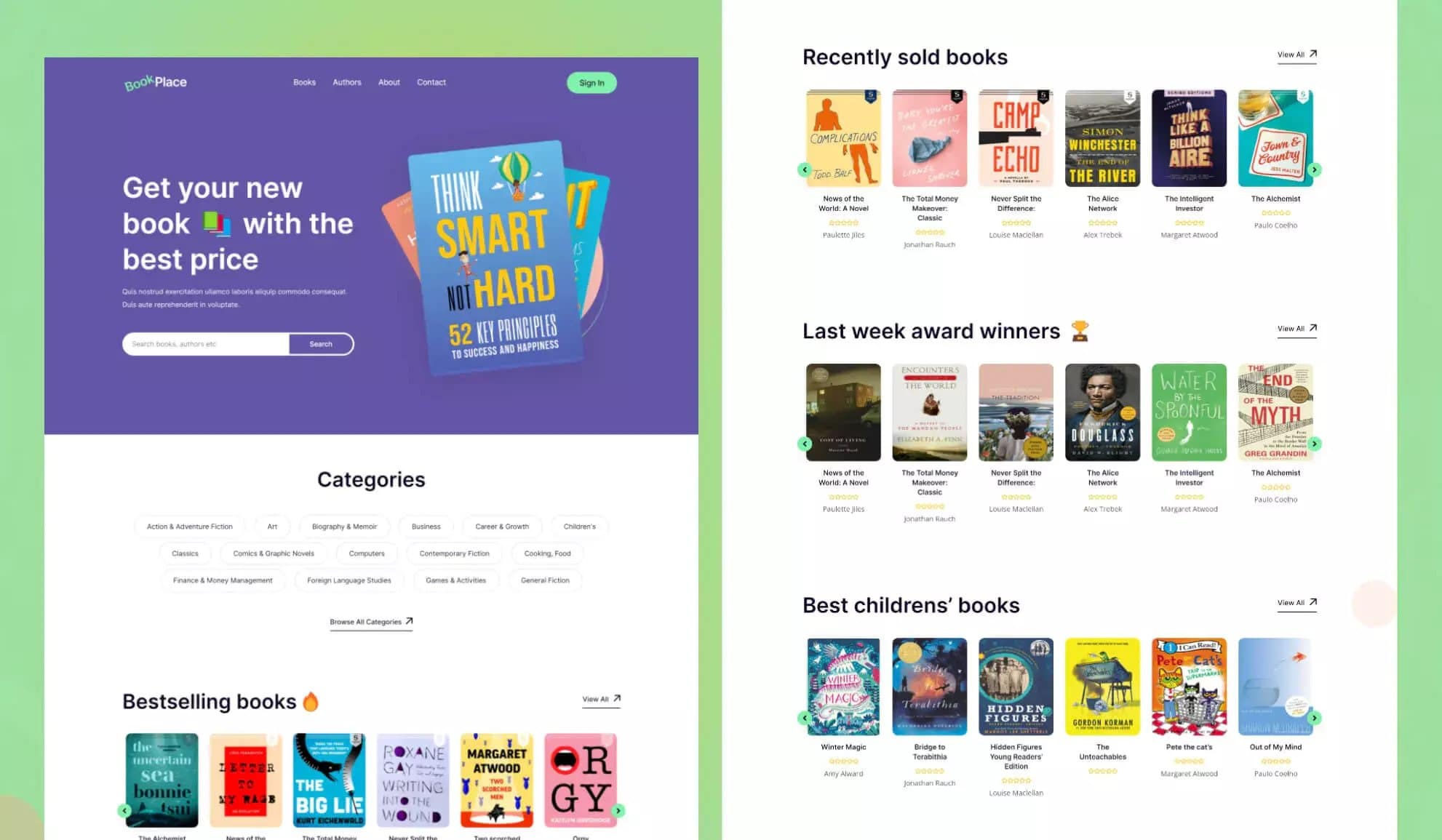The image depicts a detailed screenshot or mock-up of the "Book Place" website, seamlessly combined into a single view by dividing and aligning the content into two columns. The website features a prominent green and purple color scheme, with a purple header that reads "Get your new book with the best price." On the left column, the top left shows the "Book Place" logo, followed by a search bar. The right column displays various books, with visible titles such as "Camp Echo," "The End of the Myth," "The Big Lie," and "Think Smart, Not Hard." The lower sections of the website on both columns highlight various categories and genres, although specific details are not clearly readable. Categories such as "art," "best selling books," "recently sold books," "last week award winners," and "best children's books" are mentioned. The overall layout is user-friendly, showcasing book titles and covers in an organized format, making it easy for users to explore different genres and new releases.